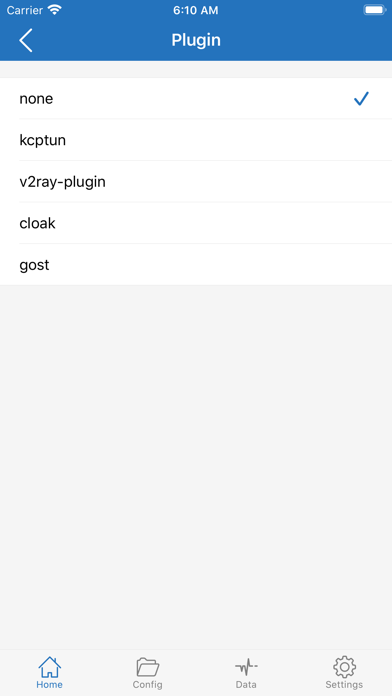### Descriptive Caption

This screenshot depicts the options menu for a plug-in configuration on a mobile device. At the very top, the status bar displays a carrier signal, a Wi-Fi icon, the time "6:10 AM," and a full battery indicator, all against a blue background. On the left side of this bar is a back arrow next to the label "Plug-In."

The main section of the screen features five plug-in options listed in black lowercase text. The first option, labeled "none," is marked with a blue checkmark on the right, indicating it is currently selected. The following options are labeled "KCPTUN," "V2RAY-plugin," "cloak," and "GOST," respectively.

The background of this section is predominantly white, devoid of any separating lines. At the bottom of the screen, four icons are aligned in a row: a blue house icon labeled "home," a gray folder icon labeled "config," a heart monitor line icon labeled "data," and a gear icon labeled "settings."

There is no additional context to explain the function of these plug-ins, and the user is unfamiliar with the frameworks mentioned.